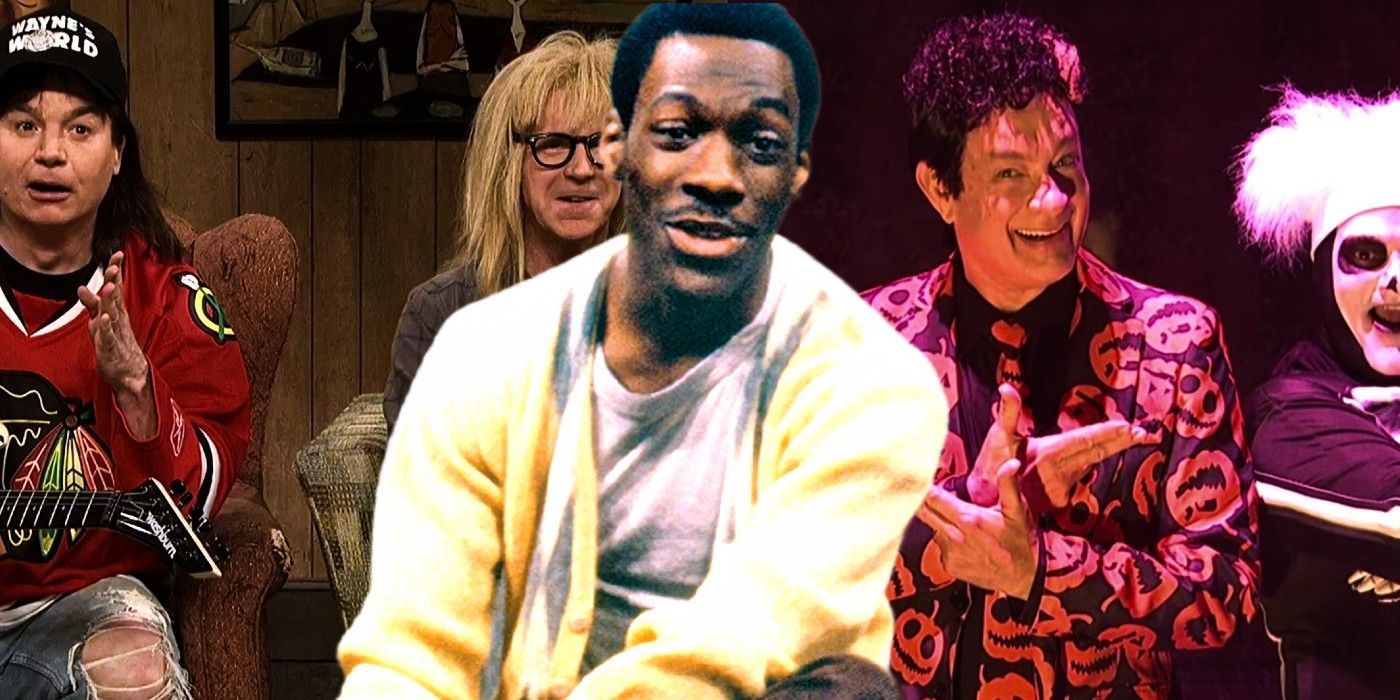The image is a detailed, composite Photoshop creation featuring several iconic actors and characters from "Saturday Night Live." At the center of the image is Eddie Murphy, seemingly portraying his Mr. Robinson character, in a yellow sweater over a white shirt, mid-speech with his mouth open. To Eddie Murphy's left are Mike Myers and Dana Carvey as their "Wayne's World" characters, Wayne and Garth. Myers sports a black "Wayne's World" cap, a red Chicago Blackhawks jersey, and torn blue jeans, sitting on a red chair, while Carvey, with long blonde hair and black-rimmed glasses, grins from a yellow checkered sofa. The background is a wood-paneled wall featuring a picture of at least two people, one with crossed arms.

To the far right in the image, Tom Hanks is dressed as David S. Pumpkins, complete with a black suit adorned with jack-o'-lanterns, a pumpkin necktie, and a black shirt. He has curly hair with a white streak and is making a gun-like gesture with his hands near his chest, smiling. Adjacent to Hanks is one of his skeleton dancers, identifiable by their black, skeletal bodysuit with a white-painted face, black lips and eye circles, and white fuzzy hair. Each actor and character in this artistic creation was digitally inserted, never having actually posed together in real life, emphasizing the seamless Photoshop collage of these beloved "SNL" personalities.